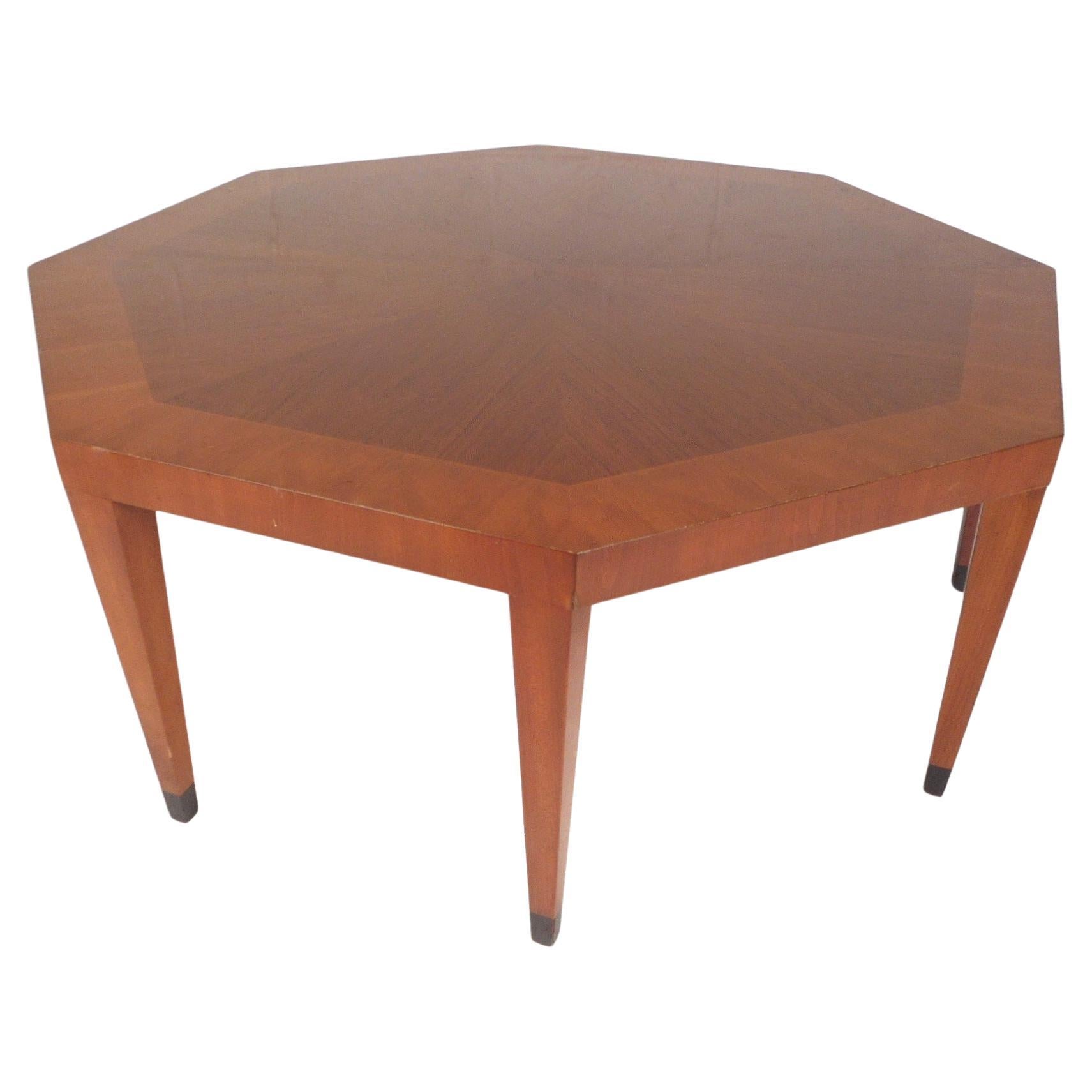This image is a detailed, color photograph with a white background, showcasing an octagonal wooden coffee table. The table, which dominates the picture, has eight sides and features a striking design. The center consists of eight triangular pieces of darker wood, likely walnut, arranged with their pointed tips converging to form an octagonal shape. The table's border is made of lighter, reddish-brown wood, resembling cherry, and displays a subtle gradation with a herringbone pattern around the edges. The table's legs, matching the cherry wood border, taper down to brass caps, with the very ends painted black, giving them a distinctive look. The image presents a clear, unobstructed view of the top and front portions of the table, highlighting its intricate wood grain and craftsmanship. The overall style is photographic representational realism, emphasizing the table's detailed and realistic appearance.